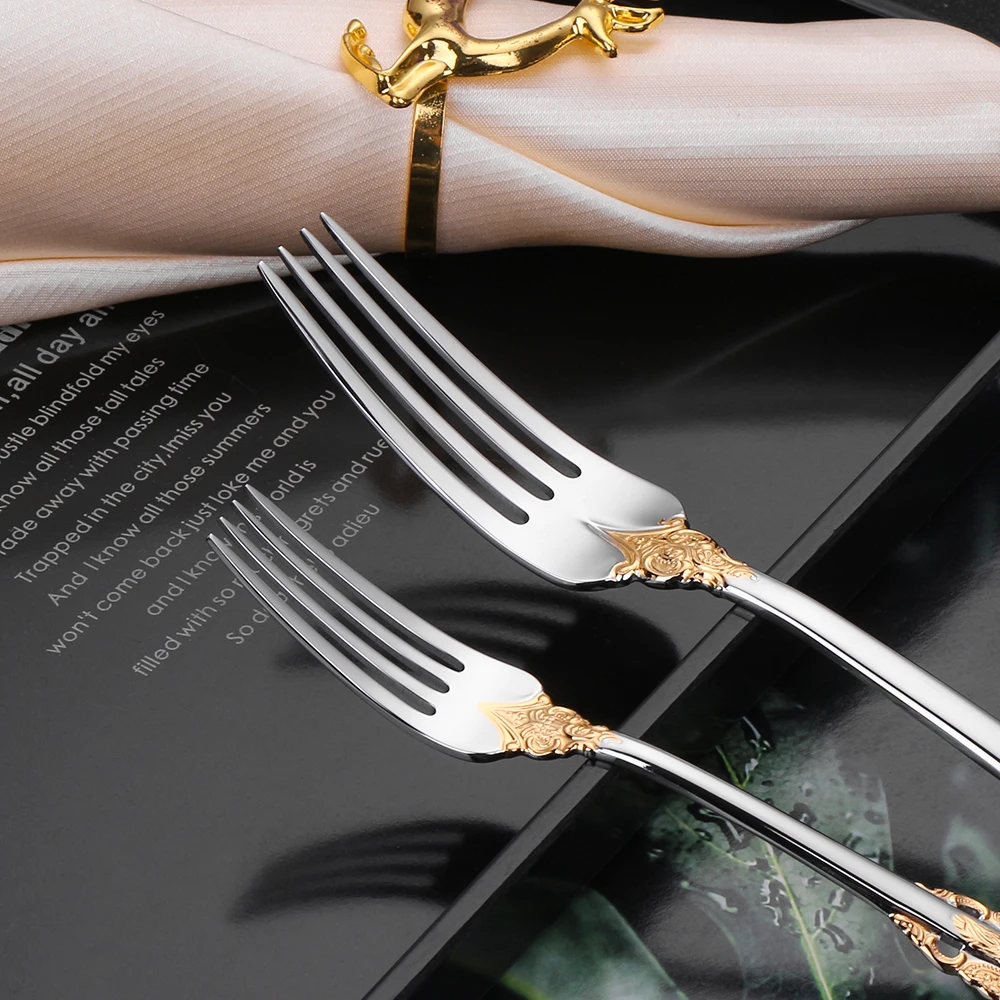This image is a detailed, artistic photograph featuring two ornate forks laid out on a stylishly designed table setting. The primary focus is on the forks, which are silver with intricate gold engravings near the base and the end of the handles, giving them an elegant appearance. The fork on the left is slightly smaller than the one on the right, both featuring four tines that converge into a triangular tip. Below these forks, there is a black, framed piece of poetry, partially obscured but visible enough to read lines like, "All day, blindfold my eyes... Trapped in the city, I miss you." The tray or mat beneath has a leafy print design adorned with water droplets. At the top, there's a rolled-up, slightly peach-colored napkin secured by a gold napkin ring with a deer motif. This setup appears meticulously crafted, likely for an artistic display or to showcase the forks in a fashionable manner.